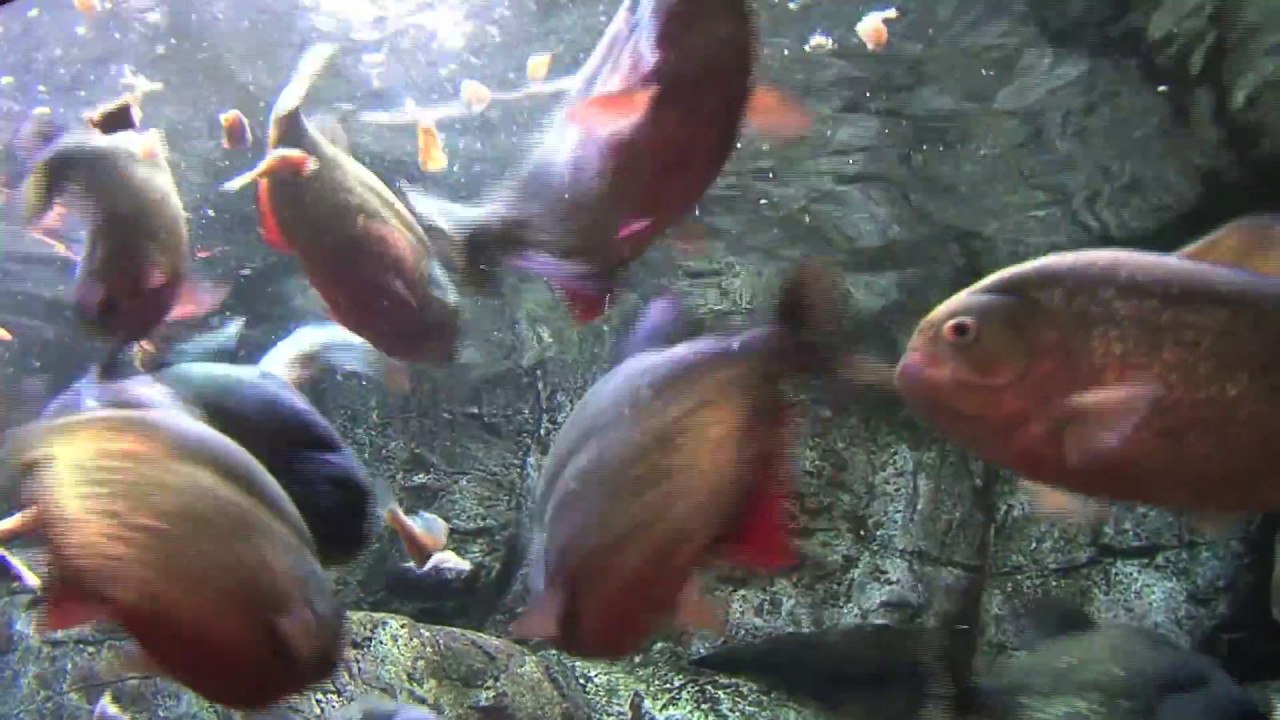The underwater photograph captures a dynamic scene of several fish swimming energetically in a clear body of water. The image is characterized by sunbeams filtering from the top, illuminating the entire shot and creating a beautiful interplay of light. The backdrop features large gray and white rocks towards the bottom half of the photo. In the foreground, seven to eight medium-sized fish with grayish and reddish tones swim in various directions, creating a blur of motion. One fish, notably to the right, appears to be looking directly at the camera, its eye and fins clearly visible. The overall scene is lively, almost as if the fish are in a feeding frenzy, with tiny specks of food floating around. The detailed close-up showcases the fish’s large mouths and eyes, capturing the underwater world's vibrant and bustling atmosphere.